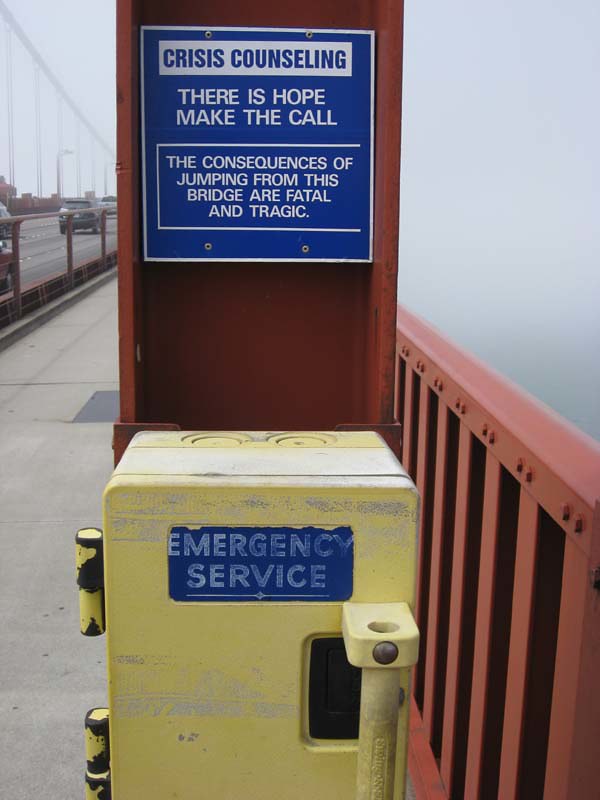The image captures a somber scene set on a busy bridge with a cement walkway adjacent to a road crowded with cars. The bridge is bordered by terracotta-colored metal railings on the right side, beyond which a blurry expanse of the ocean is faintly visible. Dominating the foreground, a terracotta pillar supports a blue and white sign that reads, "Crisis Counseling: There is hope. Make the call. The consequences of jumping from this bridge are fatal and tragic." Below this message, attached to the pillar, is a yellow emergency service box with a blue label, likely containing a phone or button to call for help. To the left of the walkway, an emergency service station stands, featuring a yellow box at the front and a taller brown shelf at the back, further emphasizing the gravity and importance of the support available to those in distress.